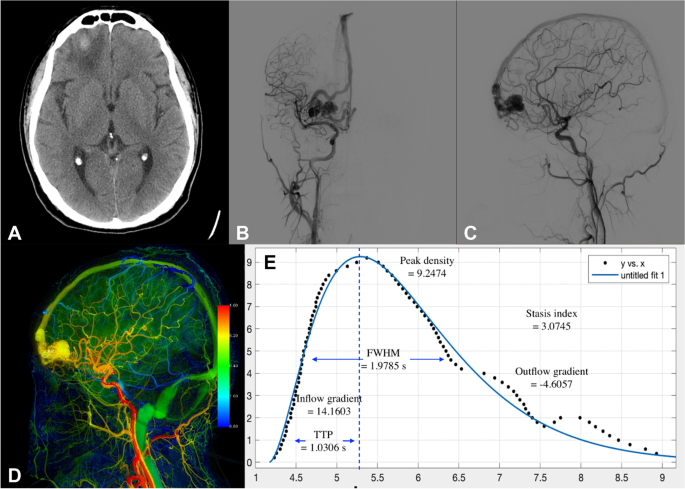The compilation of images displays various types of medical imagery and graphs related to brain analysis, labeled A through E. Image A appears to be either a CT or MRI scan of the brain, predominately normal except for some black shading in the very front part, suggesting a potential brain bleed or stroke. Images B and C reveal the intricate vasculature of the brain, possibly from an angiogram, depicting the veins without showing brain matter. Image D is a vibrant, neon-colored depiction of the brain, likely highlighting nerves or electrical activity. Image E features a hyperbolic graph discussing metrics such as inflow gradient, peak density, stasis index, and outflow gradient, which pertain to blood flow within the brain.